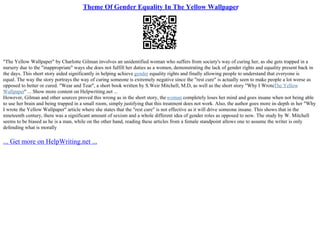The image is a small and detailed screenshot from a website centered on the theme of gender equality, specifically discussing "The Yellow Wallpaper." At the top, there's a blue hyperlink labeled "Theme of Gender Equality in The Yellow Wallpaper," suggesting it leads to more information. Below this, there's a QR code framed in standard black-and-white square patterns, typically scanned with an iPhone or Android device. The screenshot contains two paragraphs of tiny, black text that are difficult to read. At the bottom, another blue hyperlink reads "Get More on HelpWriting.net," indicating it directs users to additional writing resources on that site.